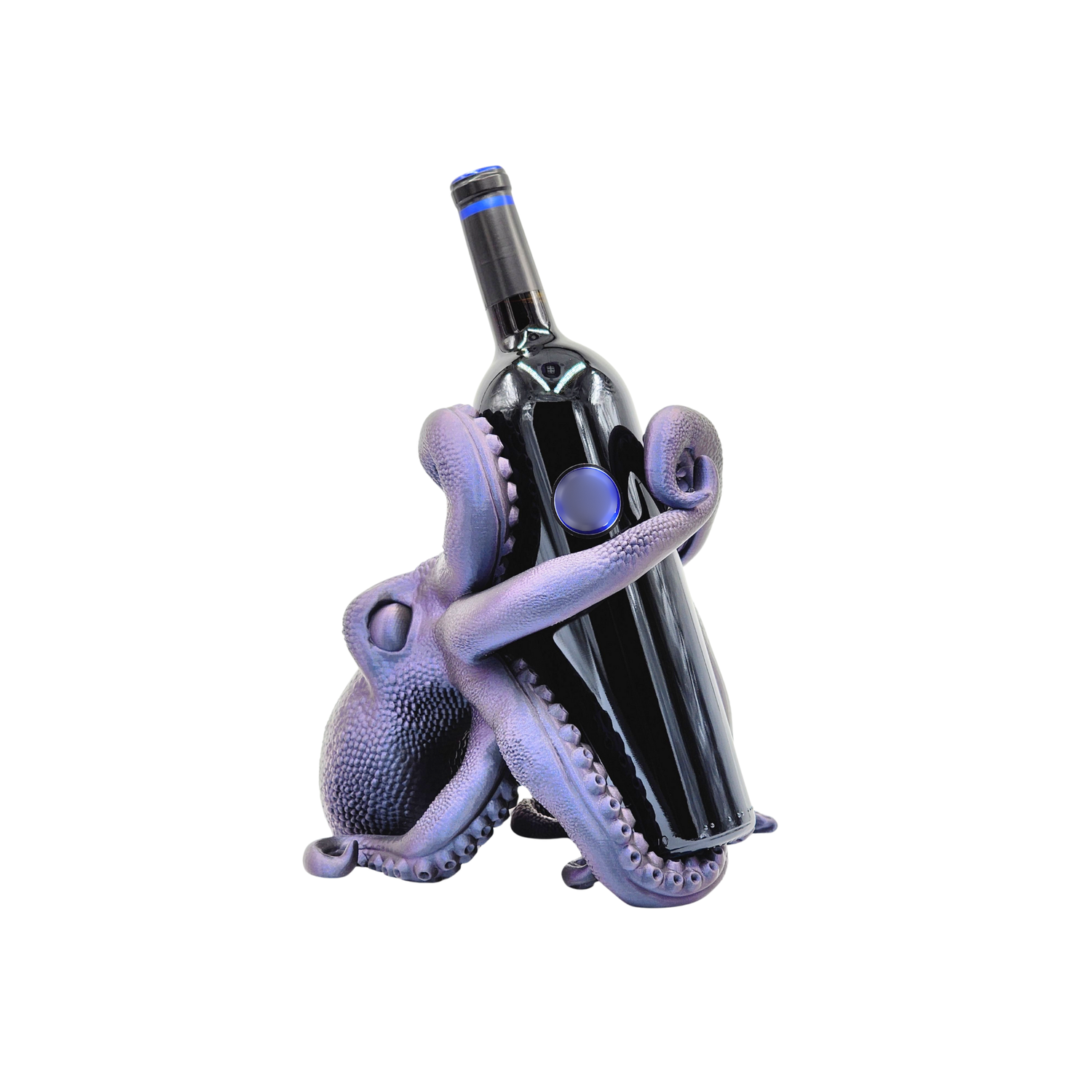This image depicts a unique, detailed, and iridescent light purple octopus wine bottle holder positioned in the bottom left corner against a white background. The octopus is on its side with its head pointing to the left and its tentacles artistically wrapped around a long black wine bottle. Its eyes, which are a darker shade of purple, face upward, and its textured skin with scaly and reptile-like features can be seen. The octopus's tentacles display visible suckers and intricate movements: one tentacle wraps around the neck of the bottle, another curls underneath its head to the left, while others interlock around the bottle, showcasing the octopus's secure grip. The wine bottle itself is slightly tilted to the left, featuring a blue circle in the center along with a silver cap and a thin blue line encircling the neck. The image emanates a sense of artistic elegance and functionality, highlighting the octopus's detailed craftsmanship.